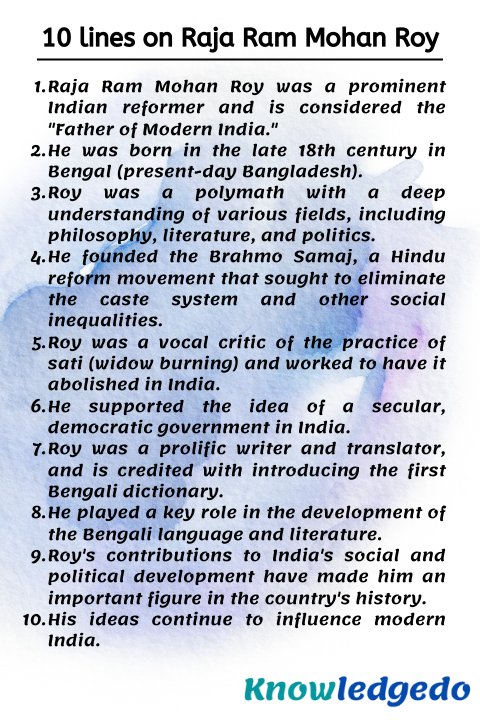**Screenshot Description:**

In this image, we see a partial screenshot of a website, focused on a small segment at the lower right-hand corner. The text elements within the image suggest educational content. One notable element is the website's presumed name or a portion of it, where the partial word "acknowledged" is visible, albeit with the final "O" appearing slightly separated, suggesting that the actual site name might be longer. The "no" in "acknowledged" stands out in an aqua blue font, while the rest of the letters, including the final "O," are in medium blue.

The content of the screenshot is laid out within a rectangular area featuring a subtle, watercolor-like background with shades of blue and lavender, lending a gentle aesthetic to the display. The primary text is in a black font, making it easily readable against the light background. Dominating the top of the content is a headline in bold black that reads, "10 Lines on Raja Ram Mohan Roy" – with the name carefully spelled out as "R-A-J-A, R-A-M-M-O-H-A-N-R-O-Y" to aid accuracy.

Below this headline, the screenshot details a list of 10 lines, which are neatly numbered, summarizing the life and contributions of Raja Ram Mohan Roy. The first line introduces Raja Ram Mohan Roy as a prominent Indian reformer and acknowledges him as the "father of modern India." The remaining lines continue to provide a succinct biography of this historical figure.